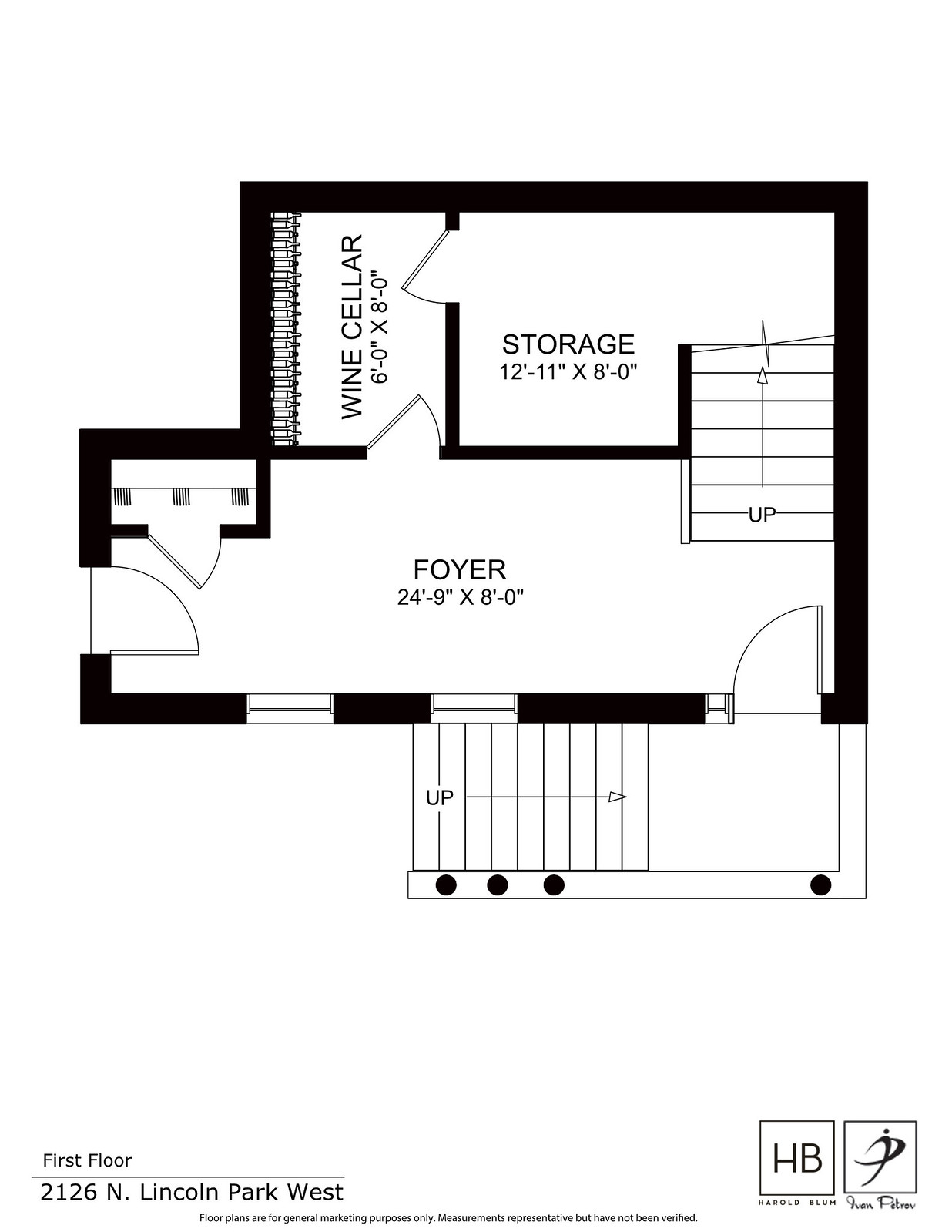This is an intricately detailed illustration designed to educate viewers about various areas within the depicted space. At the very back, you'll find the labeling for a "Wine Cellar" marked with dimensions "6'-0" x 8'-0", highlighted in black text. Adjacent to that, on the right, there is a disjointed black line surrounding the label "Storage" with dimensions "12'-11" x 8'-0". A dense grouping of lines follows, where the term "Up" is indicated, guiding the eye downward to a designated "Foyer" area marked "24'-9" x 8'-0". This "Foyer" is the largest space visually characterized by a long white rectangular shape bordered in black. Beneath this section, you'll notice elongated rectangular shapes accompanied by the word "Up" alongside a right-pointing arrow. Additionally, three filled-in black dots appear below this area, leading to some informational text positioned at the bottom left of the illustration. This text indicates "First Floor" and notes the location as "21-26 North Lincoln Park West."